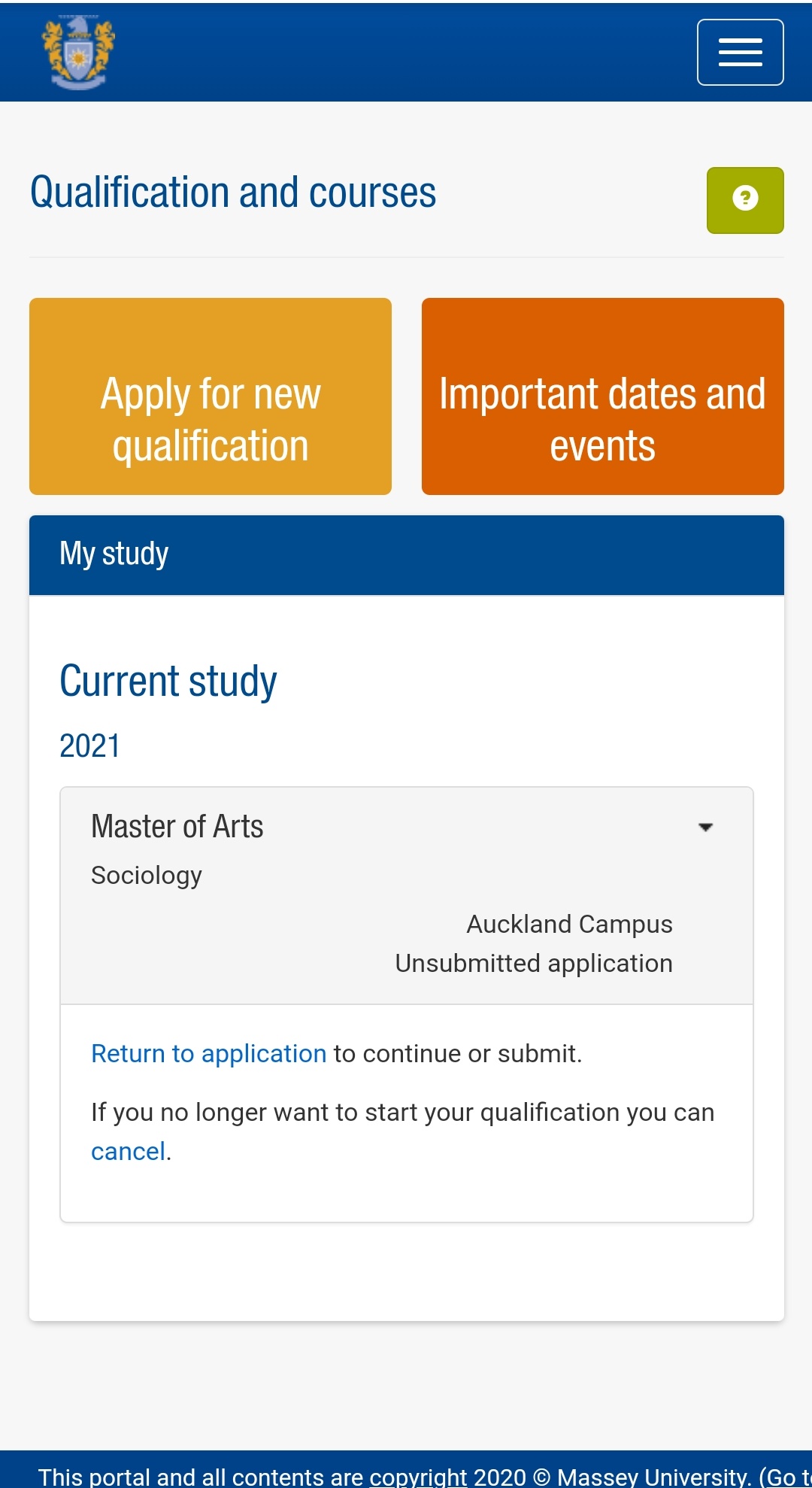The image displays a screenshot of a website interface, possibly formatted for a mobile phone. At the top, a blue band spans across the screen, featuring a grey and orange shield logo flanked by orange decorative scrolls on either side. To the far right, there is a white hamburger menu icon. 

Below this top section, the primary background is white, adorned with blue and black text. The section begins with the label "Qualifications and Courses" written in blue. Adjacent to this is a green button displaying a white circle with a question mark inside.

Further down, there is an orange rectangle on the left side with white text that reads "Apply for New Qualification." Next to it, a slightly darker orangey-red rectangle displays "Important Dates and Events." The orange shade on the left has a more yellowish hue, while the one on the right leans towards a reddish tone.

Following this, another blue band appears with "My Study" written in white. Below it, on a white background, "Current Study" in blue is labeled for the year 2021. Underneath, in black text, it details a "Master of Arts, Sociology, Auckland Campus," marked as an unsubmitted application. Positioned just above this description on the right side is a small down arrow. Below this, blue text prompts the user to "Return to application to continue or submit." If the user no longer wishes to start the qualification, they are given the option to "Cancel" in blue text.

All of this information is contained within a large square bordered at the top by a blue band. At the bottom, there is a slightly darker greyish background, featuring another blue band with white text. It states, "The portal and contents are copyright 2022, Copyright Massey University." The text near the bottom edge appears cut off, with only the partial characters "GE" visible, indicating that this portion of the text is likely truncated.

Overall, the interface is organized into sections defined by color bands and buttons, making it user-friendly and easy to navigate.